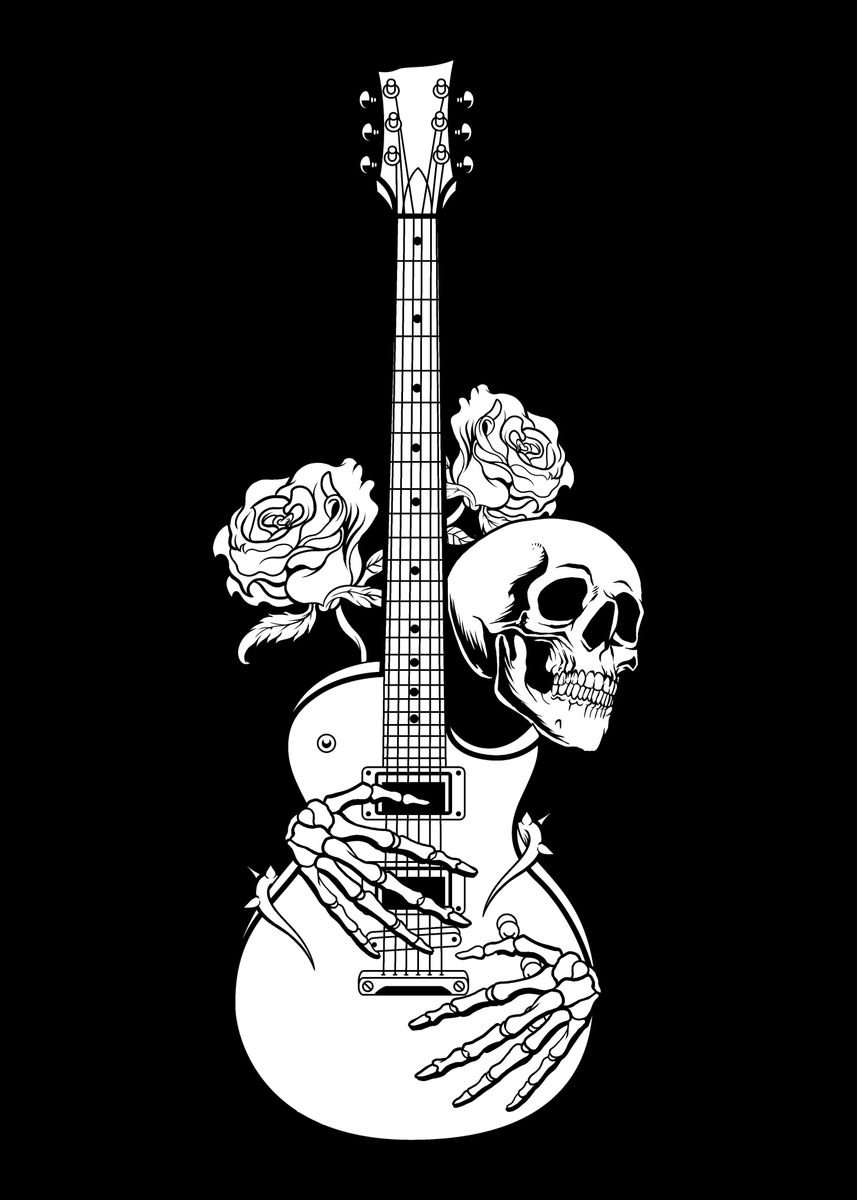In this black and white graphic image, the background is completely black, highlighting a stark and simple art style. An electric guitar stands upright in the foreground, embraced by a human skeleton. The skull, positioned to the right of the guitar, appears to be looking into the distance. The skeletal hands cradle the guitar, with bony fingers wrapping around the body and neck of the instrument. Two roses are prominently featured, one positioned above the skull and another near the neck of the guitar, their thorny vines meandering around the guitar's shape. The image captures a haunting yet elegant scene with its monochromatic tones, focusing on the interplay between the skeletal figure, the guitar, and the delicate roses.